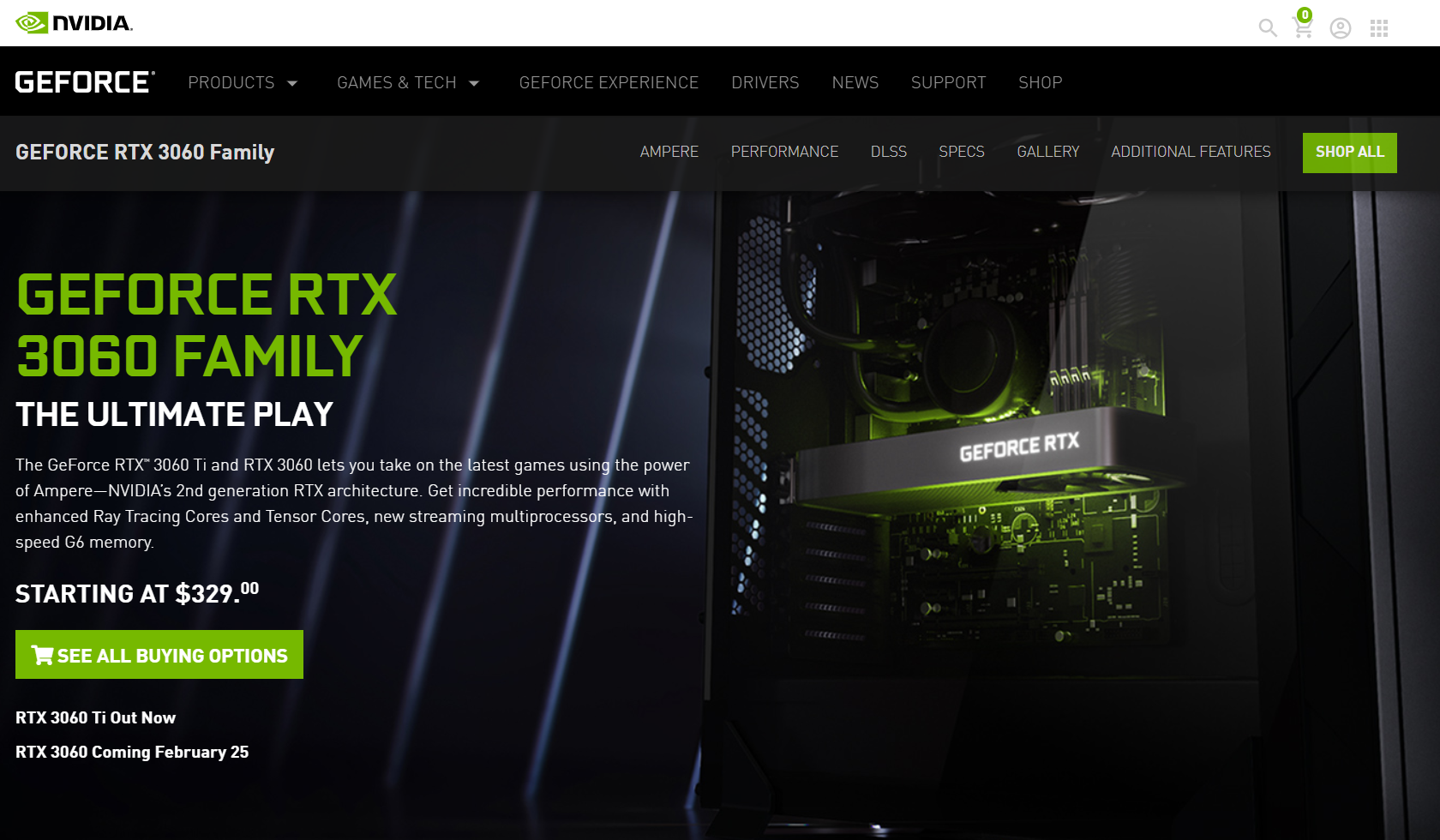The image features a detailed layout that begins with a top header set against a white background. Towards the upper left of the header, an icon appears as a green rectangle with a stylized, slanted E in white; the middle part of the E is designed as a swirl. To the right of this icon, "NVIDIA" is prominently displayed in black lettering. Below this, a section with a black background contains the label "GEFORCE" in a digitized white font with a trademark or registered symbol positioned to the upper right of the E.

Following this section, a main menu is present, showcasing several options in uppercase thin gray lettering: "Products," "Games," "Tech," "GeForce Experience," "Drivers," "News," "Support," and "Shop." Both "Products" and "Games" feature gray downward-pointing arrowheads, indicating expandable submenus. 

Beneath the header is a subheader area. To the left, bold white capital lettering announces "GEFORCE RTX 3060," followed by "Family" with only the F capitalized. Adjacent to this on the right, another menu appears in light gray capitalized thin lettering, maintaining the digitized aesthetic. This menu lists: "Ampere," "Performance," "DLSS," "Specs," "Gallery," and "Additional Features." Lastly, to the far right, there is a lime green rectangular icon that contains the text "Shop All" in bold white lettering.